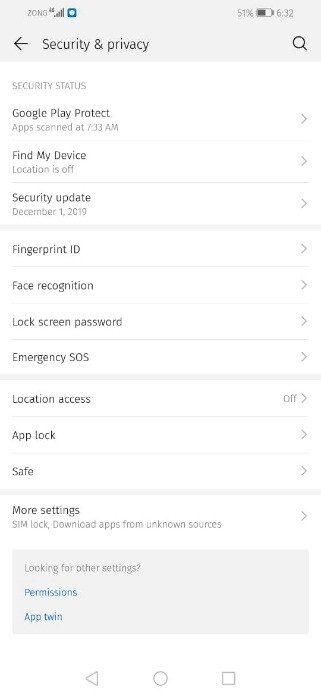Screenshot from an Android device displaying the "Security and Privacy" settings page. The battery level is at 51% and the time is 6:32 AM. The "Security Status" section shows Google Play Protect with the last app scan performed at 7:33 AM. Below that, "Find My Device" is highlighted with the location turned off. The security update is dated December 1st, 2019. Other security features listed include "Fingerprint ID," "Face Recognition," "Lock Screen Password," "Emergency SOS," "Location Access" (off), "App Lock," and "Safe," with each option accompanied by a right-facing caret indicating expandable menus. At the bottom of the page, there is a prompt: "Looking for other settings?" followed by two hyperlinks: "Permissions" and "App Twin."